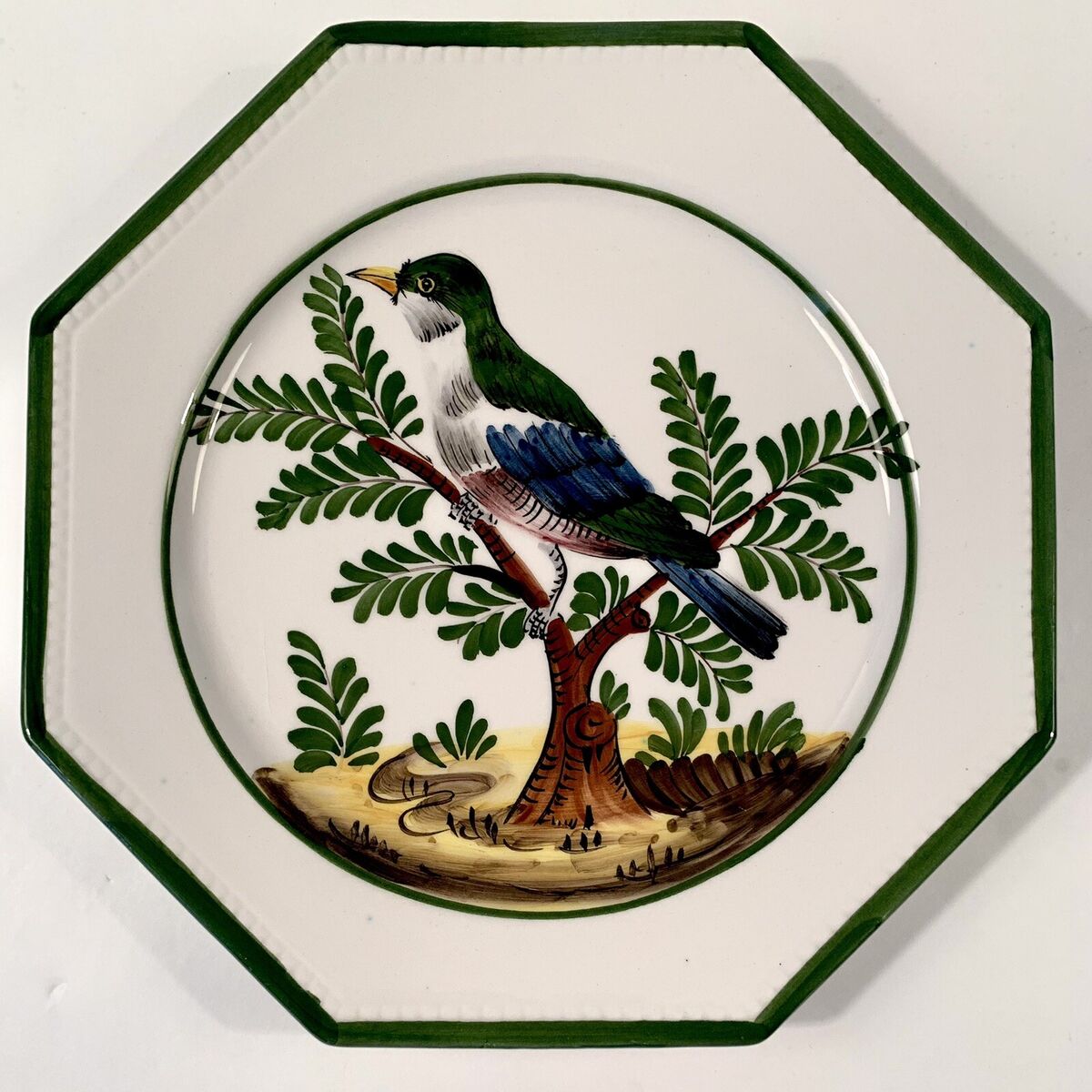This image showcases a decorative serving plate set against a white background. The plate is octagonal in shape and features a dark green border along its edge. Made from refined China, the plate has a central circular green border that encircles a detailed painting. The artwork depicts a blue and white bird with a red underbelly, a yellow beak, and white and black striped legs. The bird is perched on a brown tree trunk adorned with green leaves. Surrounding the tree are green bushes and tan ground with brown swirls and lines that add texture. Just inside the plate's green border, there's a delicate pattern of little lines. The plate casts a shadow to its right side on the white surface.